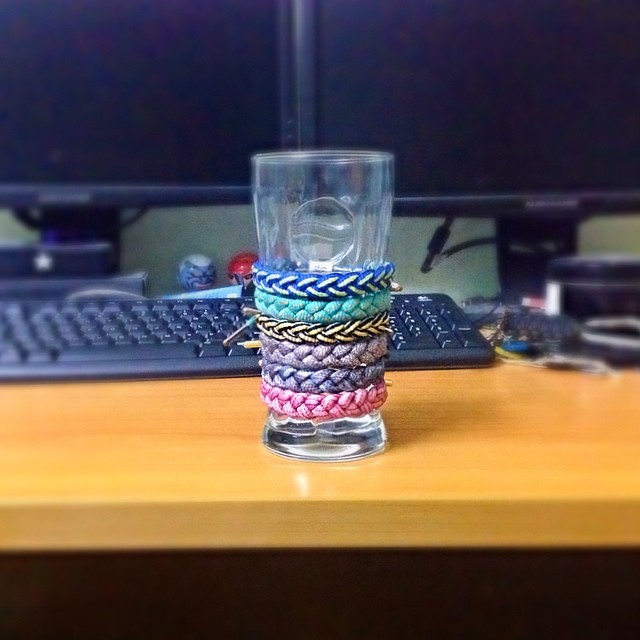In this detailed photograph, a clear glass cup prominently features the Pepsi logo—minus the iconic colors—set meticulously on a light brown wooden desk. Surrounding the cup are six distinct woven wristbands in quartered patterns and varying hues: the topmost is navy blue, followed by one in teal, another in black and yellow, then a purple wristband, a darker purple one, and lastly, a medium pink. The unusual detail of the undone edges and metal tips, typical of shoelaces, suggest a braided design for each piece. The desk also hosts a black gaming keyboard, and in the background, two Alienware gaming monitors stand guard, each adorned with a small figurine—one blue and white, the other red. The scene blends elements of gaming and personal style, capturing a slice of life at a well-used workspace.